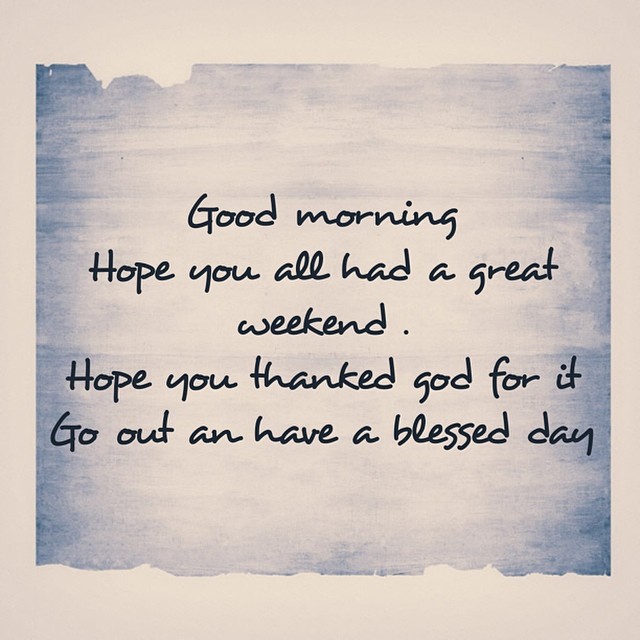The image is a square poster-style quote with a beige border surrounding a blue square that mimics the look of a torn piece of paper. The blue background varies in shade, with darker blue along the rough, torn edges at the top and bottom, and a lighter, almost sky-like blue streaked with white at the center, creating a radiant effect. Centered within this blue area is the quote, written in a black, handwritten-style font: "Good morning. Hope you all had a great weekend. Hope you thank God for it. Go out and have a blessed day."